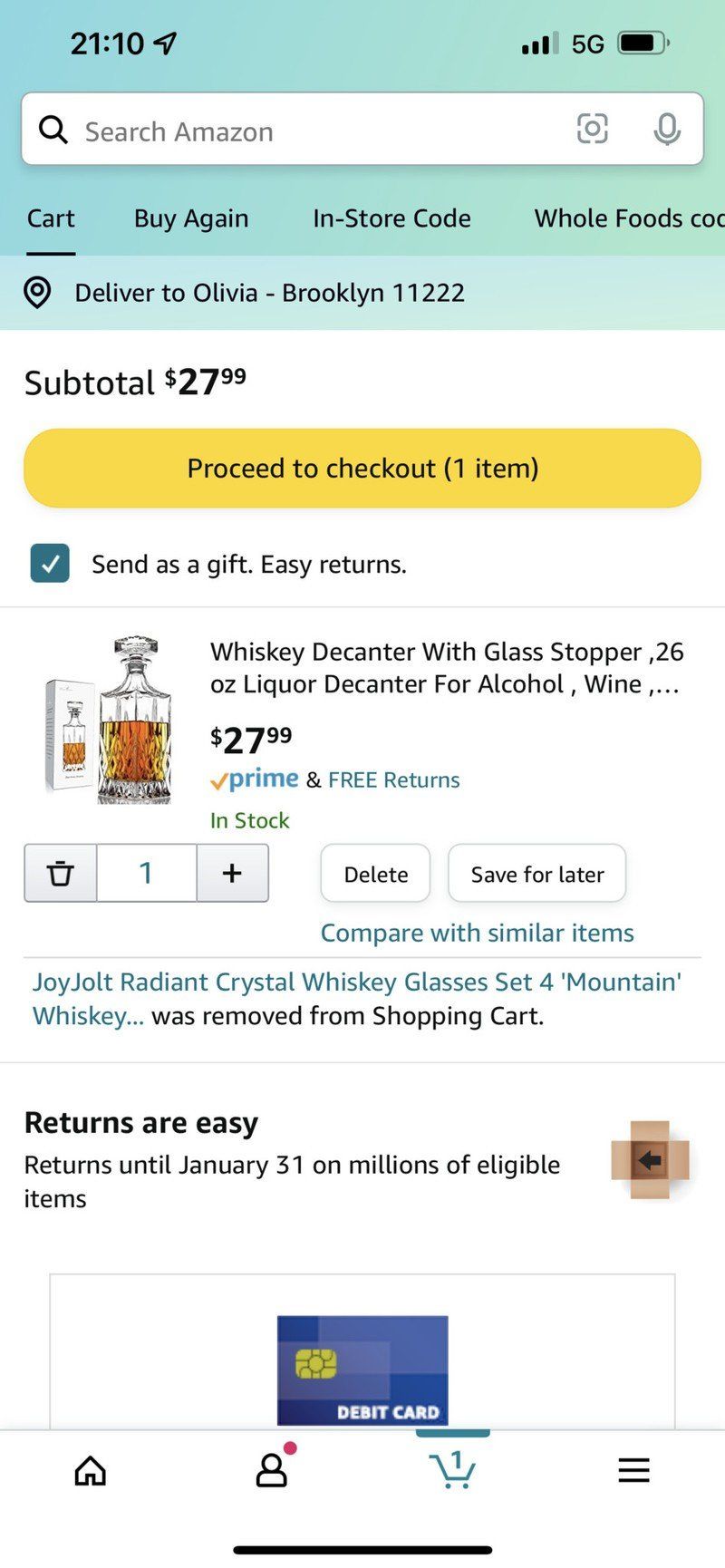The image captures an Amazon web page displayed on a smartphone screen. At the top of the screen, there's a "Search Amazon" header with a white search box set against a light green background. Tabs are positioned near this search box, providing different navigation options.

Immediately below the search box, several quick-access options are listed: "Cart," "Buy Again," "Install Code," and "Whole Foods." An address bar beneath these options displays the delivery address: "Deliver to Olivia, Brooklyn, Leaven, 2222."

The main content area is predominantly white with black text. Here, it lists the subtotal amount, "$27.99," and features a prominent yellow button with black text that reads, "Proceed to checkout (1 item)." A checked checkbox below this button indicates, "Send as a gift, easy return."

The page then highlights the product: a "Whiskey Decanter with Glass Dropper, 26-ounce Liquid Decanter for Alcohol," priced at $27.99. Accompanying the product description on the left is an image of a transparent glass filled with brown wine. Additional options such as "Quantity: 1," "Delete," and "Save for later" are provided alongside the product details.

Further down, there is a section titled "Compare with similar items." Underneath this section is a notification about a removed item: "Joy Jolt Aurora Crystal Whiskey Glasses Set for Mountain Whiskey was removed from shopping cart."

At the bottom of the page, a blue card is visible with "Debit Card" written on it. Footer navigation options include buttons for "Home," "Profile," "Cart," and "Options." Additionally, a note mentions the flexibility of returns: "Returns are easy; returns until January 31 on millions of eligible items."